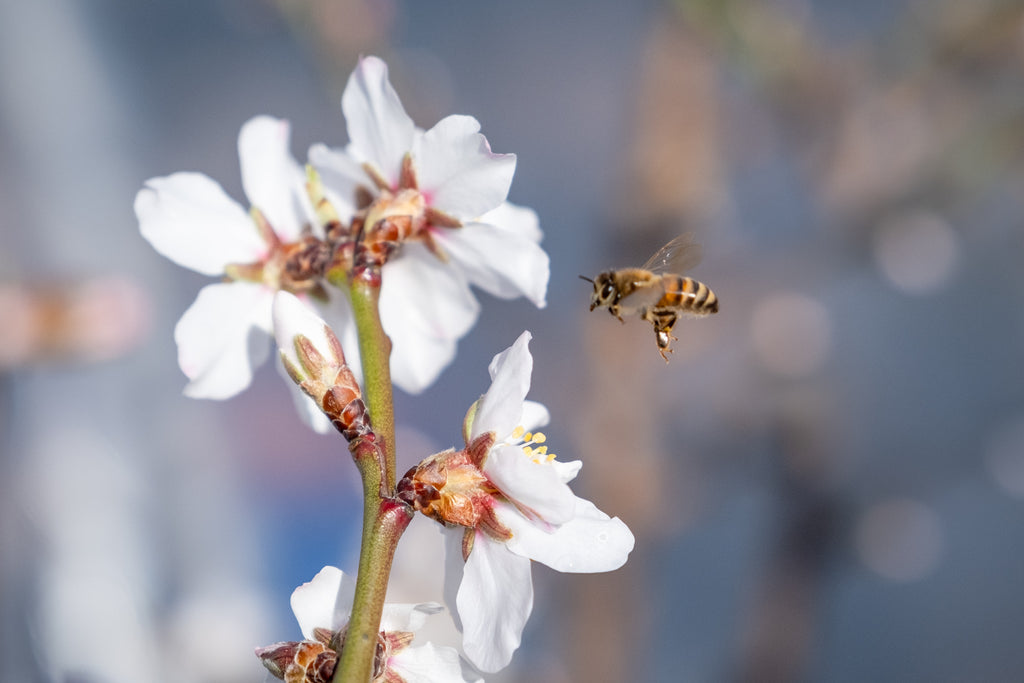This image captures a honeybee poised to land on one of four white flowers that emerge from a single green stem. The flowers are characterized by reddish-brown bases, and their interiors feature yellow stamens, particularly prominent in the bottom right-hand corner, where the bee appears to be heading. The honeybee, distinguished by its goldish-yellow body adorned with black stripes, has yet to collect any pollen on its legs but seems moments away from doing so. The bee's delicate wings and furry upper body are visible against the soft, blurry backdrop, where subtle hints of muted blues and beige create a pleasing bokeh effect. This artistic background ensures that the focus remains squarely on the interaction between the bee and the flowers, drawing the viewer's eye to the intricate details and the imminent pollination process.